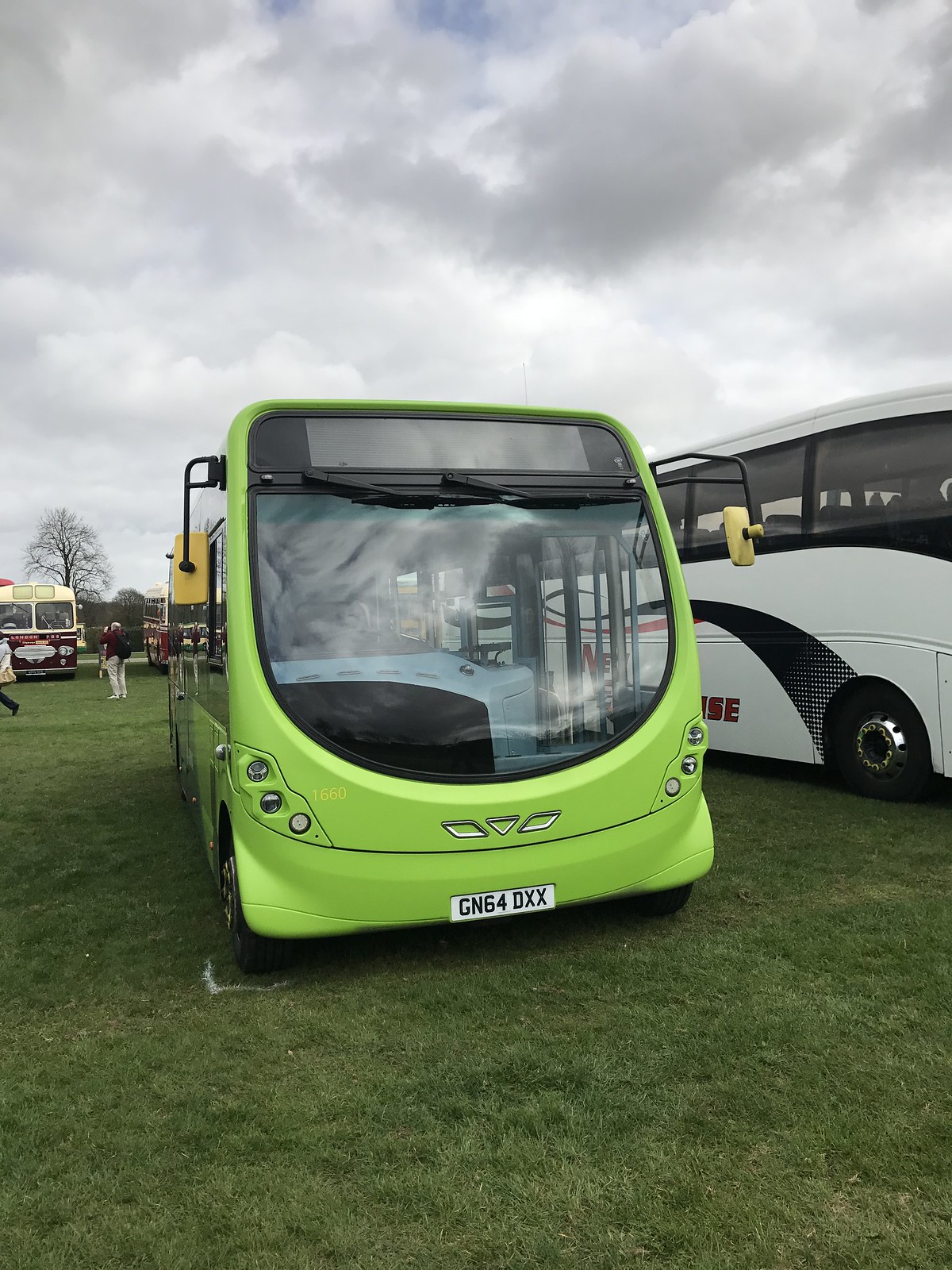In the foreground of the image, a vibrant lime-green transit bus is parked on lush green grass, showcasing a striking, futuristic design. The bus's expansive, teardrop-shaped windshield nearly extends to the bumper, flanked by yellow wing mirrors and a structured, angular emblem at the front. Three small, diagonally positioned headlights add to its modern aesthetic, alongside two outwards-angled grille squares, divided by a centered triangle. The bus bears a white license plate with the code GN64DXX. Above the windshield, the wipers are pointed to the right, below a blank black display panel.

Adjacent to the green bus on the right, a large white coach with swirls of black and red is partially visible, revealing hints of orange stripes through the green bus's windows. To the left, beyond the lime-green bus, there's a smaller vintage bus with a burgundy bottom and cream top, attracting several onlookers who are taking photos. The backdrop of the scene features additional older buses and distant individuals, with leafless trees standing tall against a sky filled with gray and white rainy clouds.